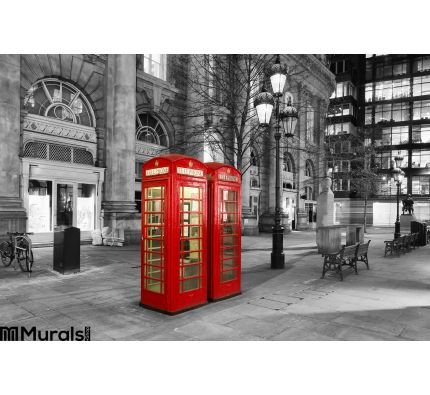This black-and-white photograph prominently features two iconic red London telephone booths in the center, their interiors warmly illuminated in yellow. These booths, positioned side by side and radiating a nostalgic charm, are the only elements in color, creating a striking contrast against the monochrome background. Surrounding the booths, one can observe the classic urban landscape comprising lampposts, street benches, and a bicycle secured to a lock area on the left side. Further back, there is a blend of architectural features, including a grand old stone building or possibly a corporate edifice, complete with abundant windows and an adjacent statue of a man, perhaps on horseback or seated. The presence of leafless trees suggests a winter setting. In the lower left-hand corner of the image, the text "MURALSII" and an 'M' logo are faintly visible, adding a hint of modern artistic branding to this otherwise timeless scene. The entire composition is devoid of people, allowing the stillness and stark color contrasts to stand out magnificently.